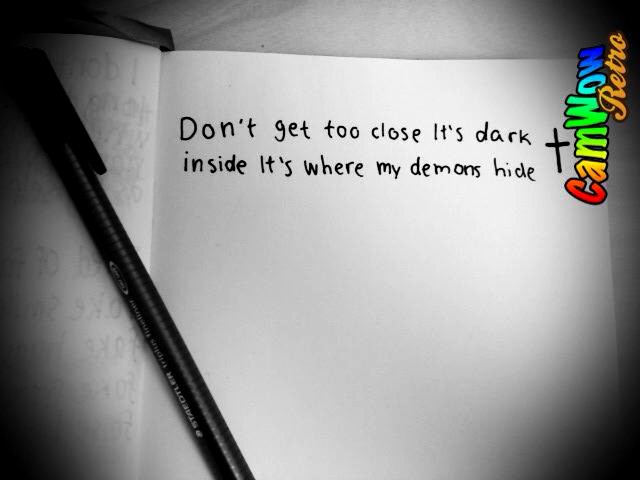The image features an open book, resembling a journal or diary, with no lines on the pages. A black pen with its lid on lies horizontally across both pages. In the top right corner, the logo "CamWow Retro" is prominently displayed in a mix of upper and lower case, starting with a red 'C,' followed by yellow 'A' and 'M' fading to green, 'Wow' transitioning from green to dark blue, and 'Retro' in an orange handwriting font, with 'R' capitalized. The corners of the photo are dark, adding a moody atmosphere. On the left page, in black text without punctuation, it says: "Don't get too close, it's dark inside, it's where my demons hide." Next to this text, a small cross is drawn, adding a personal touch. The book also features a felt fabric tassel bookmark emerging from the top center. Writing from the other side of the left page is faintly visible through the paper.